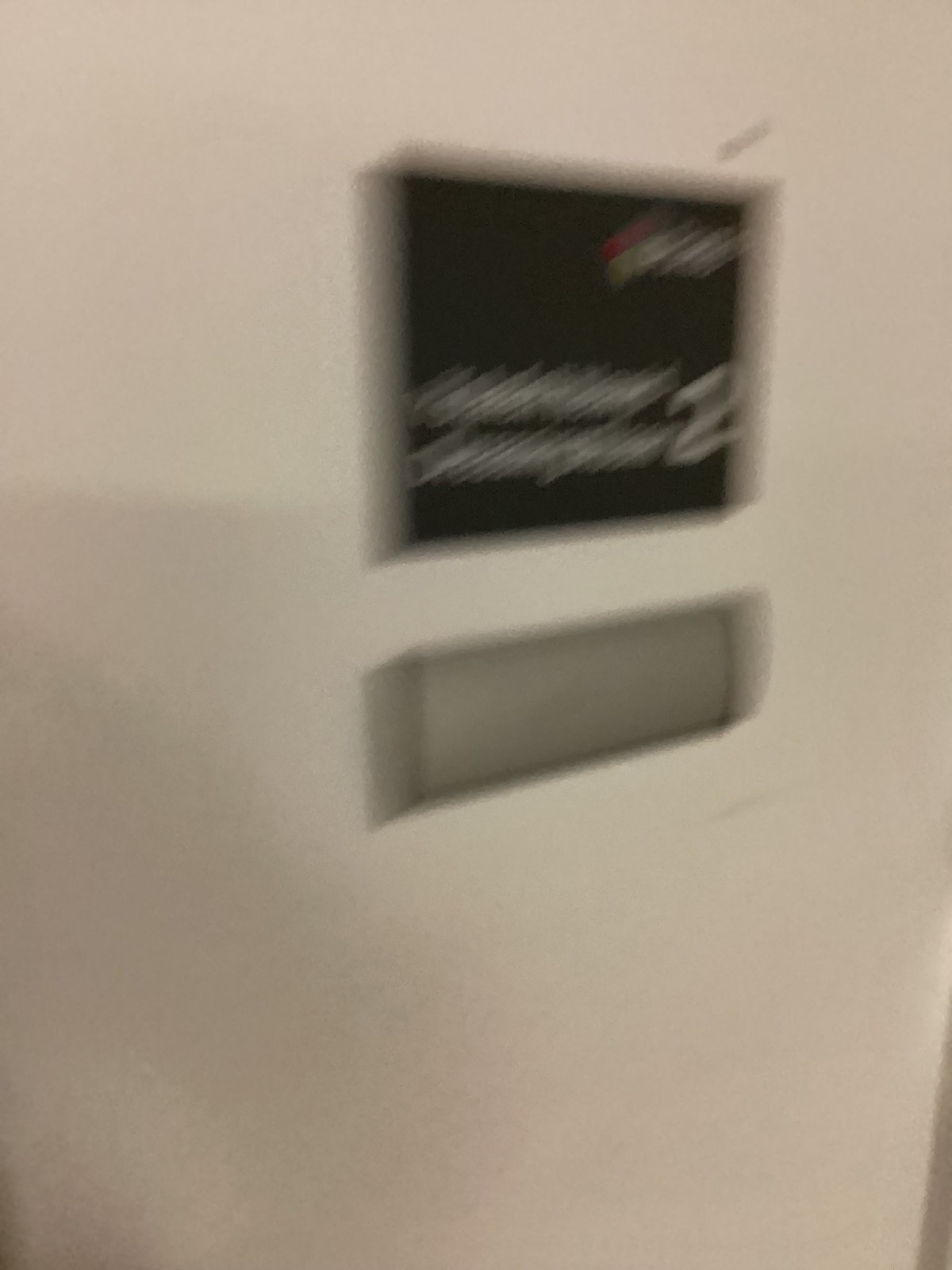This photograph depicts a very blurry scene of a white wall with some scuff marks, featuring two wall plaques. The upper plaque is a black, slightly wider-than-tall rectangle, which appears to have a red-and-white logo in the top right corner. There are two lines of text next to a partially legible number "2," though the text itself is indistinguishable due to the blur. Below this is a dark gray triangular plaque, resembling a nameplate or mail slot. The overall image gives the impression of being taken in motion, possibly by someone walking past, and includes subtle shadows on the left side, likely cast by the photographer.